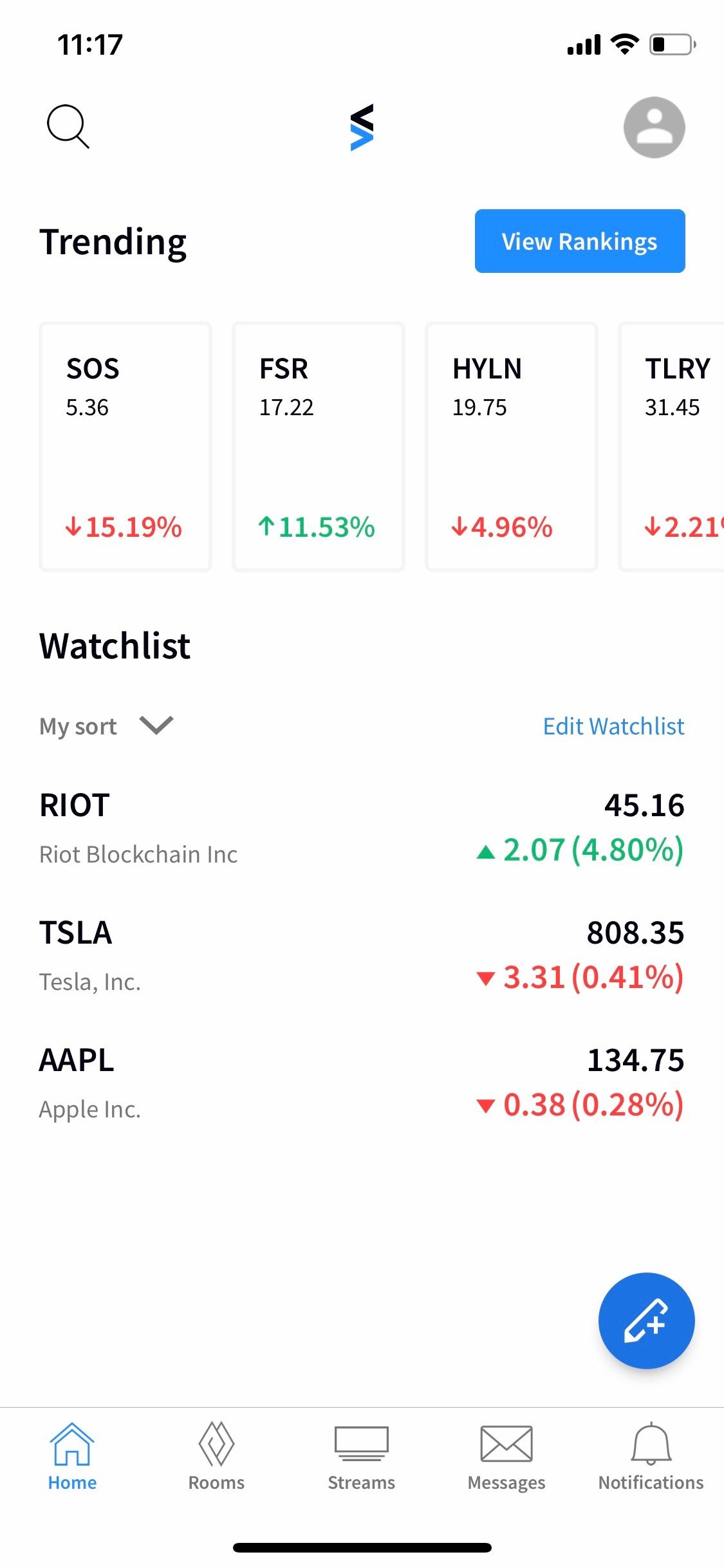This is a detailed screenshot from a tablet or smartphone. The top-left corner displays the time as 11:17 in black text. On the far right, indicators show a full network signal, full Wi-Fi signal, and a battery level at approximately one-third. Below the status bar, a magnifying glass icon is positioned to the left, followed by two arrow icons—one black arrowhead pointing left, and one blue arrowhead pointing right. Next to these is a small circle icon featuring a white silhouette of a person, likely representing a user profile.

Under this top section, the word "Trending" appears on the left in black text, and on the far right, there's a blue tab reading "View Rankings" in white text. The section below displays stock information in a tabular format:

- SOS: Priced at $5.36, decreased by 15.19%.
- FSR: Priced at $17.22, increased by 11.53%.
- HYLN: Priced at $19.75, decreased by 4.9%.
- TLRY: Priced at $31.45, decreased by 2.21%.

Further down, a "Watch List" section is shown, with options to edit and sort. The following stocks are listed:

- RIOT (Riot Blockchain Inc.): Priced at $45.16, increased by 2.07 points, equivalent to 4.8%.
- TSLA (Tesla Inc.): Priced at $808.35, decreased by 3.31 points, or 0.41%.
- AAPL (Apple Inc.): Priced at $134.75, decreased by 0.38 points, or 0.28%.